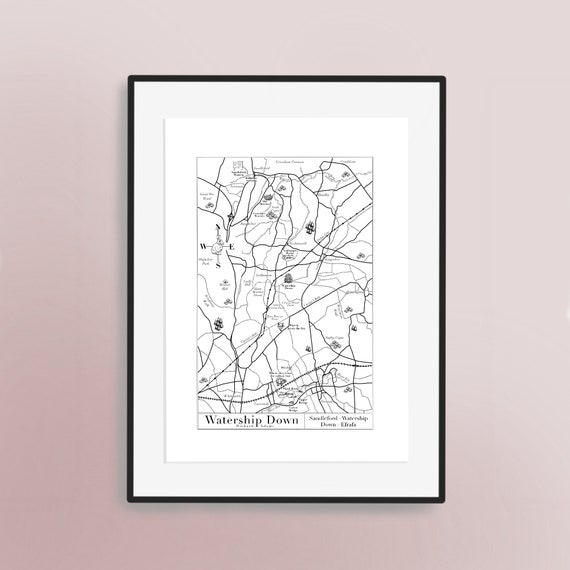This photograph captures a minimalist black and white map titled "Watership Down" mounted in a sleek, thin black frame. The map, printed on white paper, is housed within a wide white border, enhancing its monochromatic look. The frame is displayed on an off-white wall with a pinkish hue. The map itself features a series of intricate black lines, some resembling railroads and dotted pathways. A compass resides in the top left corner, guiding viewers through the depicted landscape. The title "Watership Down" is clearly marked in the lower left corner of the map, hinting at the area's layout despite the simple and clean design. The combination of the subtle wall color and the understated design of the map creates a thoughtful and aesthetically pleasing display.